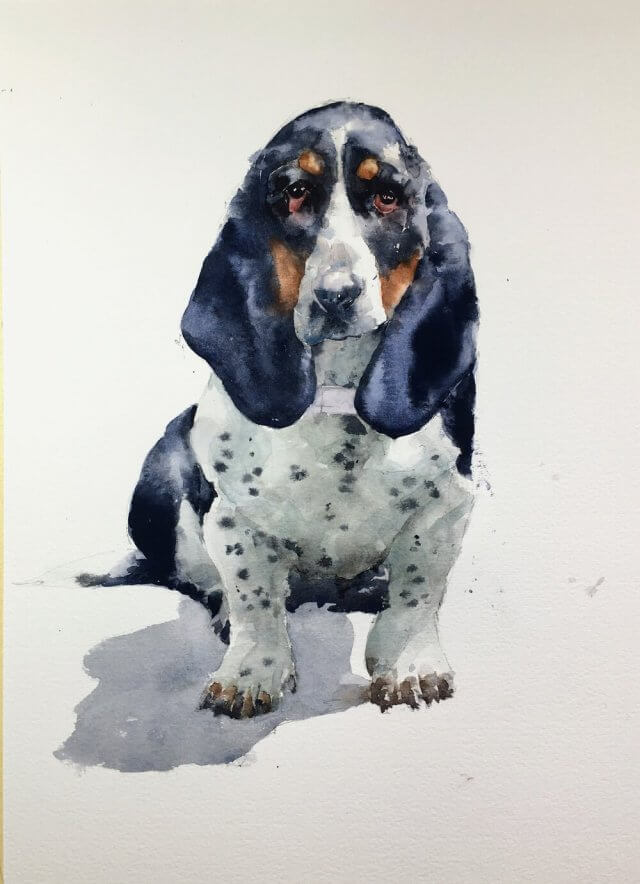This detailed watercolor painting depicts a Basset Hound with a textured, aged appearance on a whitish-gray background. The dog's distinctive features include large, long, droopy black ears and a predominantly white face with a black nose bordered by white fur. Notable details include brown spots above its eyes and on its cheeks. Its body showcases a mixture of white fur with black spots on the front legs and a black back extending towards the tail. The hound's eyes are primarily black with a hint of brown, giving them a weary expression. The painting technique allows the colors to bleed slightly, creating a soft and blurry effect that adds to the realistic portrayal despite some diffuse details. A grayish shadow beneath the dog suggests it's positioned on a white surface under strong lighting. Additionally, a subtle streak of tan adorns the left side of the painting, adding depth to the composition.